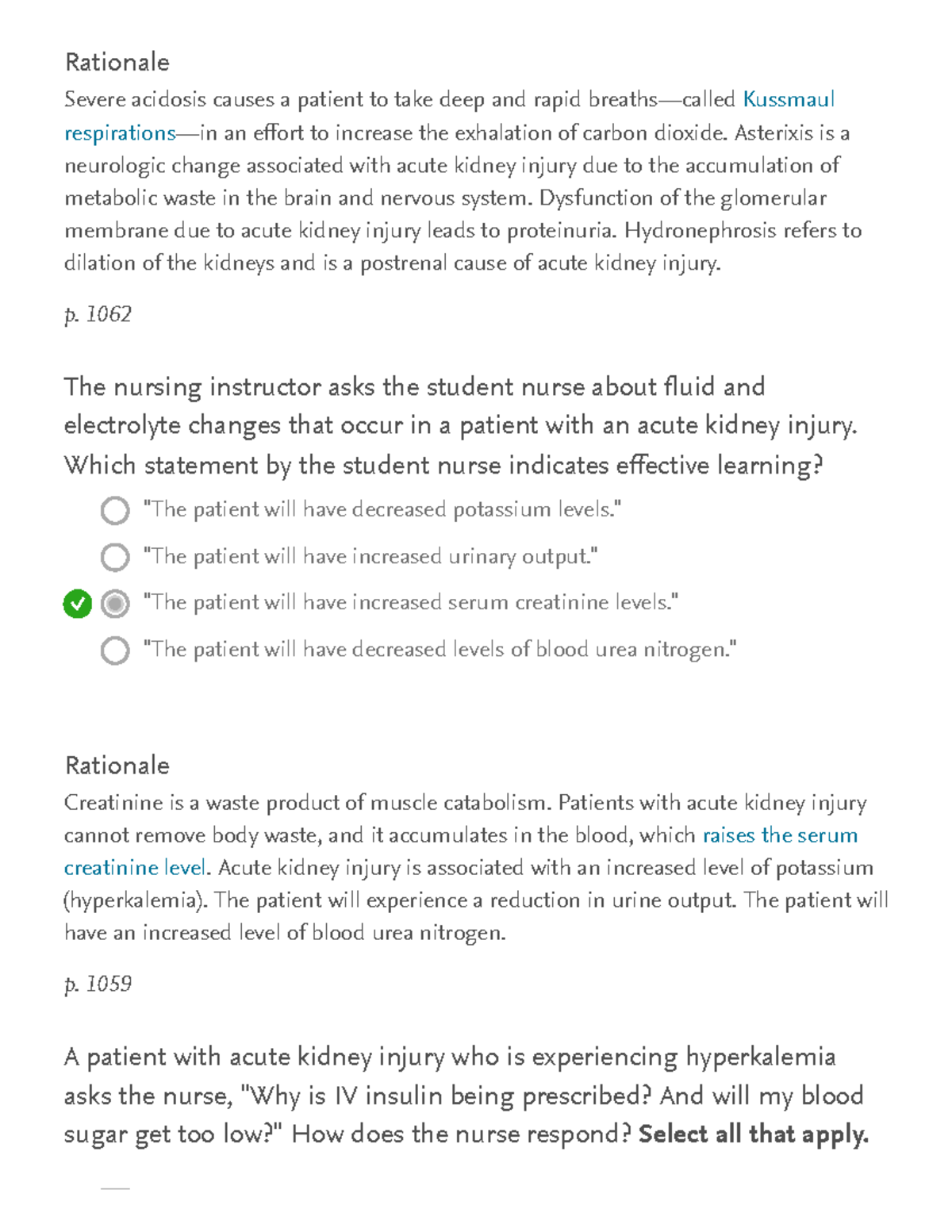The image depicts an online quiz question related to acute kidney injury (AKI) and associated pathophysiological changes. The visible text explains that severe acidosis in a patient with AKI can lead to deep and rapid breathing, known as Kussmaul respirations, as a compensatory mechanism to expel excess carbon dioxide. Additionally, neurological changes, such as asterixis, may occur due to the accumulation of metabolic waste in the brain and nervous system. The quiz also touches upon other complications of AKI, including proteinuria resulting from glomerular membrane dysfunction and hydronephrosis, a condition characterized by the dilation of the kidneys due to post-renal obstruction.

Below this explanation, the screen shows a question posed by a nursing instructor regarding fluid and electrolyte changes in patients with AKI. There are four possible answers, with the third option, "The patient will have increased serum creatinine levels," marked correct with a checkmark within a green circle. The other options include: "The patient will have decreased potassium levels," "The patient will have increased urinary output," and "The patient will have decreased levels of blood urea nitrogen (BUN)."

Further down, there is another paragraph labeled with the reference "P1059," followed by a scenario where a patient with AKI experiencing hyperkalemia inquires about the purpose of prescribed IV insulin and potential concerns about blood sugar levels. The question posed to the nurse asks how to respond, but the answer choices are not visible in the image.

This comprehensive scene highlights key concepts related to acute kidney injury for nursing students, emphasizing the importance of understanding pathophysiological mechanisms, appropriate nursing responses, and patient education.

---

This caption aims to provide a clear, comprehensive, and detailed description of the image, relevant for preparing nursing students and healthcare professionals.